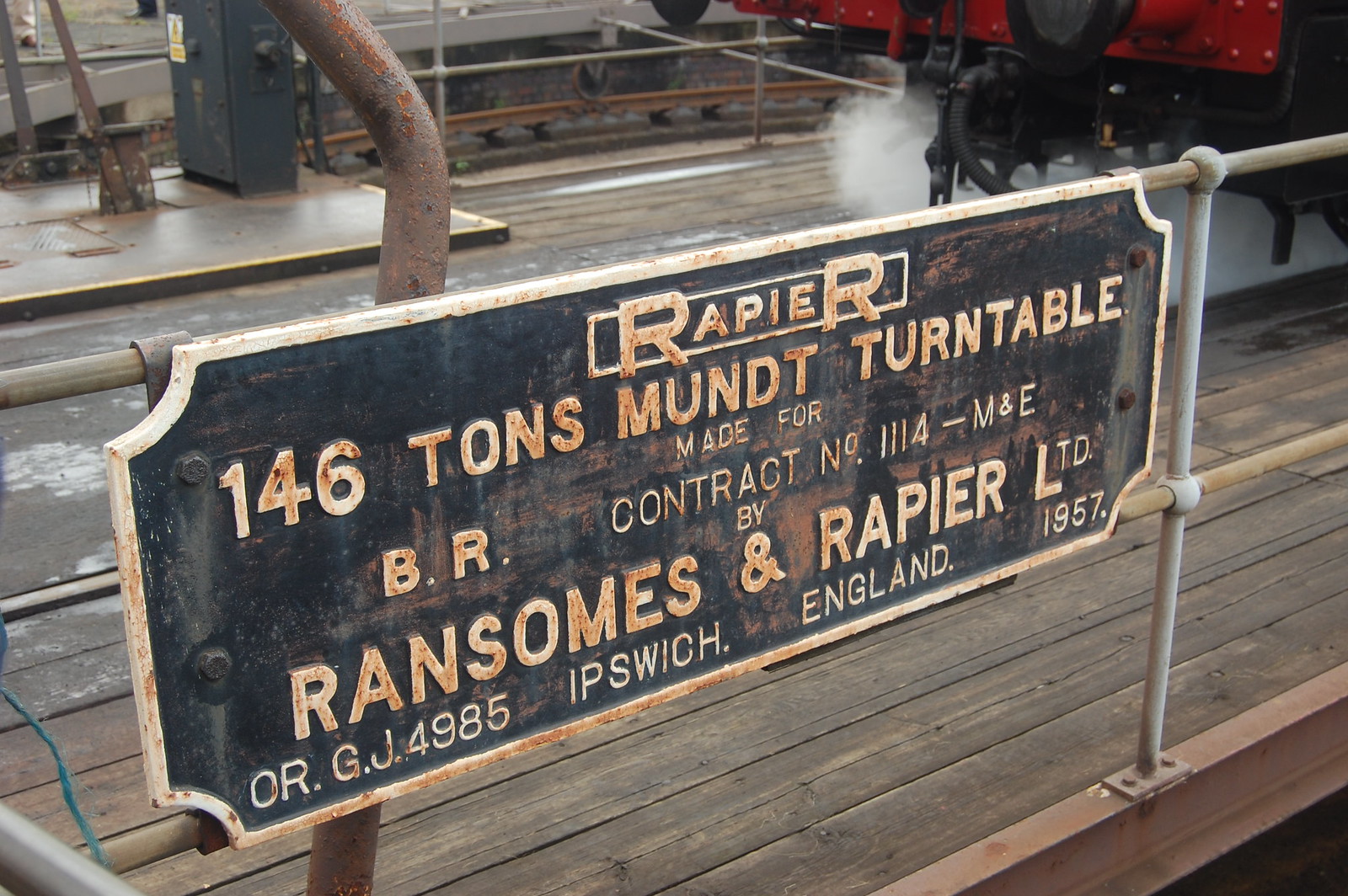The image showcases an old, weathered sign attached to a metal fence at what appears to be a train station platform. The surrounding infrastructure includes discolored brown wooden planks and rusty metal railings that frame the scene. The platform is constructed with well-used wood and metal, showing significant signs of wear and aging. In the background, numerous pipes are visible, adding to the industrial atmosphere, and there is a distant red object in the top right corner that may be a train.

The sign itself is black with a white border and white lettering, indicating its age and wear through extensive rust. The header of the sign reads "Rapier," likely the logo or company name. Below it, the text details: "146 tons, month, turntable, made for the BR contract number 1114-M&E, Ransoms and Rapier Limited, Ipswich, England, 1957." This suggests the sign references a substantial turntable used to switch train tracks, a significant piece of equipment made for a British Railways contract in 1957. The entire scene is set against the backdrop of Ipswich, England, adding historical and geographical context.